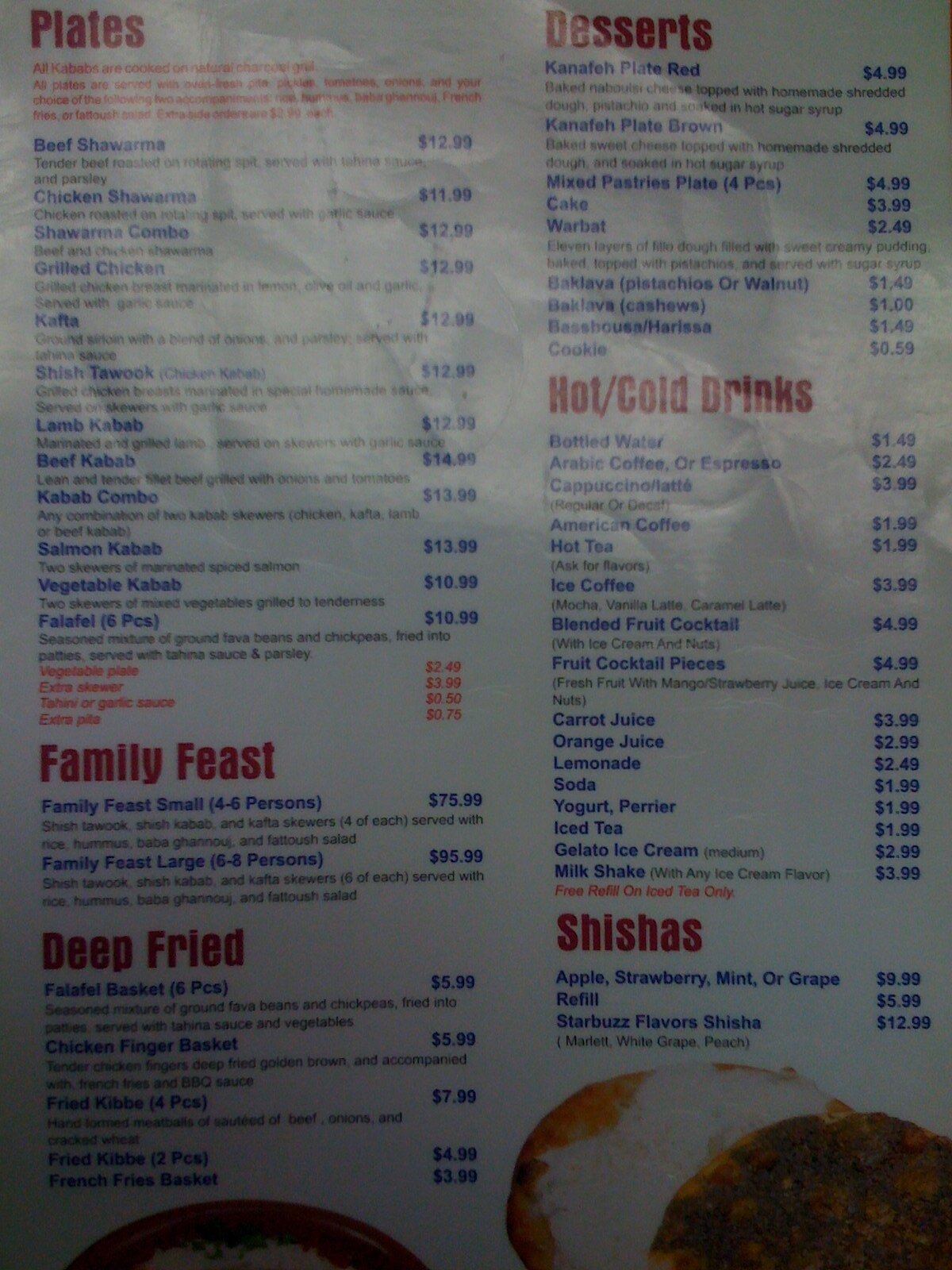This photograph depicts a menu captured under inadequate lighting conditions, creating a dim and poorly lit atmosphere. The menu, slightly curved with the top edges bending away from the camera, shows significant light reflection at its apex. The menu itself is primarily white, accentuated with red headings categorizing the different sections and additional red text indicating specific details or exceptions. Most of the text is rendered in blue across two visible columns. The headings clearly demarcate sections such as "Plates," "Family Feast," "Deep Fried," "Desserts," "Hot/Cold Drinks," and "Shishas." At the bottom of the left column, part of a round object emerges from the darkness, lacking discernible detail due to the poor lighting. Similarly, in the lower corner of the right column, an indistinct image of a food item is visible. Initially ambiguous, it appears to be either a burger or a dish accompanied by rice, though the lack of illumination obscures any defining features.